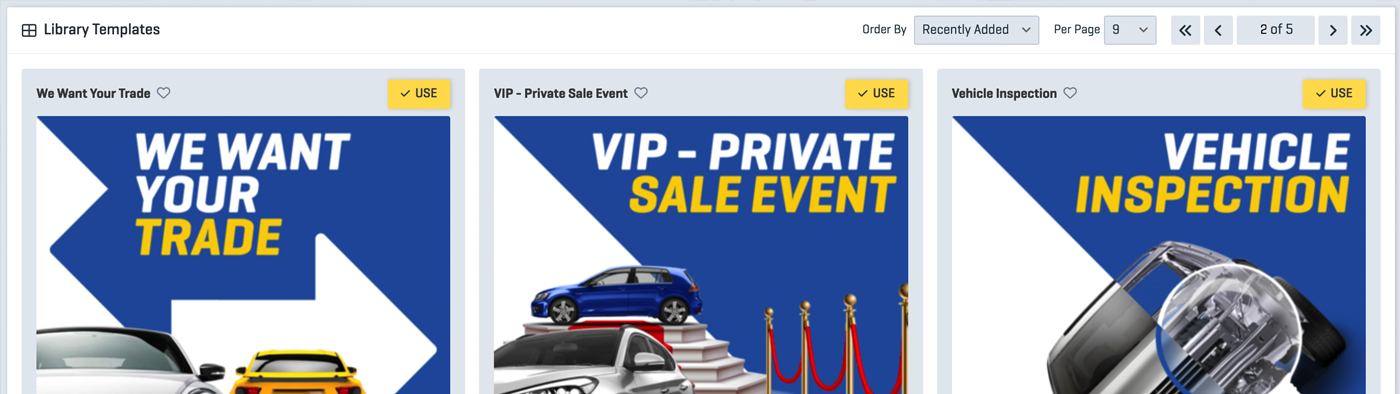This screenshot showcases the back end of a website or software interface, specifically featuring a section labeled "Library Templates" in the top-left corner. Below this label, there are three grey boxes, each containing a graphical representation for different banners. 

The leftmost box displays a banner titled "We Want Your Trade" positioned at the top left, with a prominent yellow button labeled "Use" on the right side. The corresponding image below the title features a thematic design relevant to the banner text. 

The middle box follows a similar structure, titled "VIP Privacy Element" and showing an image of a blue car. Again, a yellow "Use" button is located on the right. 

Finally, the rightmost box presents a banner with the title "Vehicle Inspection," featuring an image of a car at a diagonal angle with a magnifying glass overlay. Consistent with the others, there is a yellow "Use" button on the right side of the title.

Each banner in this section appears to be a selectable template option for use within the website or software, offering distinct visual elements and titles catered to specific functions.